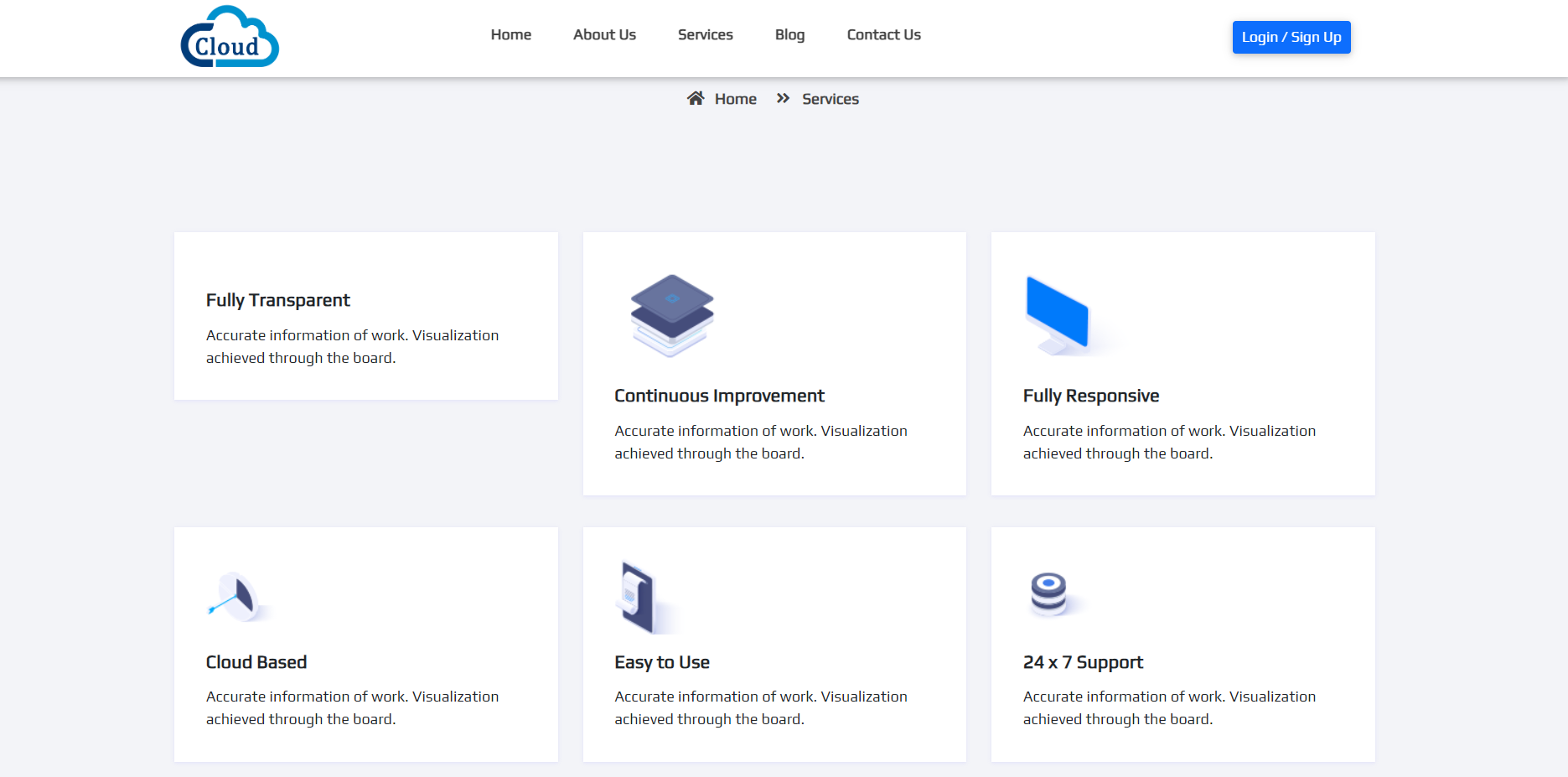In this image, the background is light blue, transitioning to white at the top where a small white cloud is surrounded by a faint blue cloud. The top section features a navigation bar with links labeled "Home," "About Us," "Services," "Blog," and "Characters," followed by blue buttons for "Login" and "Sign Up." Below this, a blue horizontal line divides the screen. Beneath the line, the page highlights navigation breadcrumbs with "Home" followed by two right arrows and "Services."

The main content area displays six white boxes, each containing unique information:

1. The first box features the text "Fully Transparent" and "Achieve through the Board" alongside an icon of blue papers.
2. The second box also states "Achieve through the Board" but focuses on "Continuous Improvement" with a blue computer screen icon marked as "Fully Responsive."
3. The third box declares "Cloud Based" with a light blue line intersecting a small blue square.
4. The fourth box emphasizes "Easy to Use," showing a blue square with white details.
5. The fifth box highlights "24x7 support," represented by a blue and white circle.
6. Throughout the design, bright blue accents are used to draw attention to key elements, ensuring the information is clear and visually engaging.